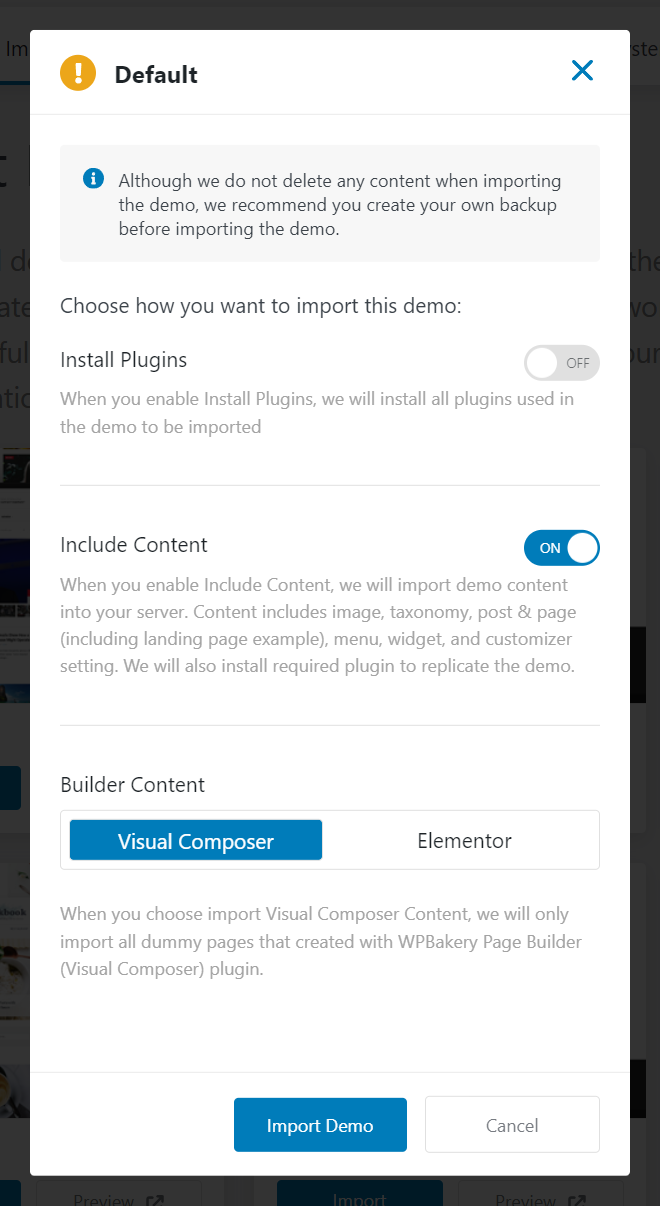This image showcases a user interface for a demo import feature, layered on top of other content with a dark gray transparent overlay. At the top of the white box, there is a mustard-colored exclamation point inside a bubble, positioned to the left of the word "Default," which is displayed in standard font. On the left side, there is a medium blue 'X' button. 

Directly below, a gray horizontal rectangular box with rounded corners contains an informational message. Within this box, there is a blue bubble housing a white eye icon. The message, written in dark gray font, advises: "Although we do not delete any content when importing the demo, we recommend you create your own backup before importing the demo."

The section beneath this message provides options for demonstration content import. It begins with "Choose how you want to import this demo."

1. **Install Plugins:** 
   - To the right, a binary option is available, with "Off" being the current selection. When hovered over, the text informs users that enabling this will install all plugins essential for the demo.

2. **Include Content:** 
   - Below, another option appears with "On" currently selected. The blue-filled bubble indicates that the option is active. It explains that enabling this will import various demo content types, including images, taxonomies, posts, pages, landing pages, menus, widgets, and customizer settings. Necessary plugins for demo replication will also be installed.

3. **Builder Content:**
   - Users have the choice between "Visual Composer" (highlighted in blue with white text) and "Elementor" (displayed in standard black text). This description elaborates that choosing to import "Visual Composer" content includes all demo pages crafted with the WPBakery Page Builder, also known as the Visual Composer plugin.

At the bottom of the interface, users are given two actionable choices:
- "Import Demo" on the left, distinguished in blue with white text.
- "Cancel" on the right, marked in a dark gray font. 

This detailed layout ensures users have clear options and information for managing their demo import process efficiently.